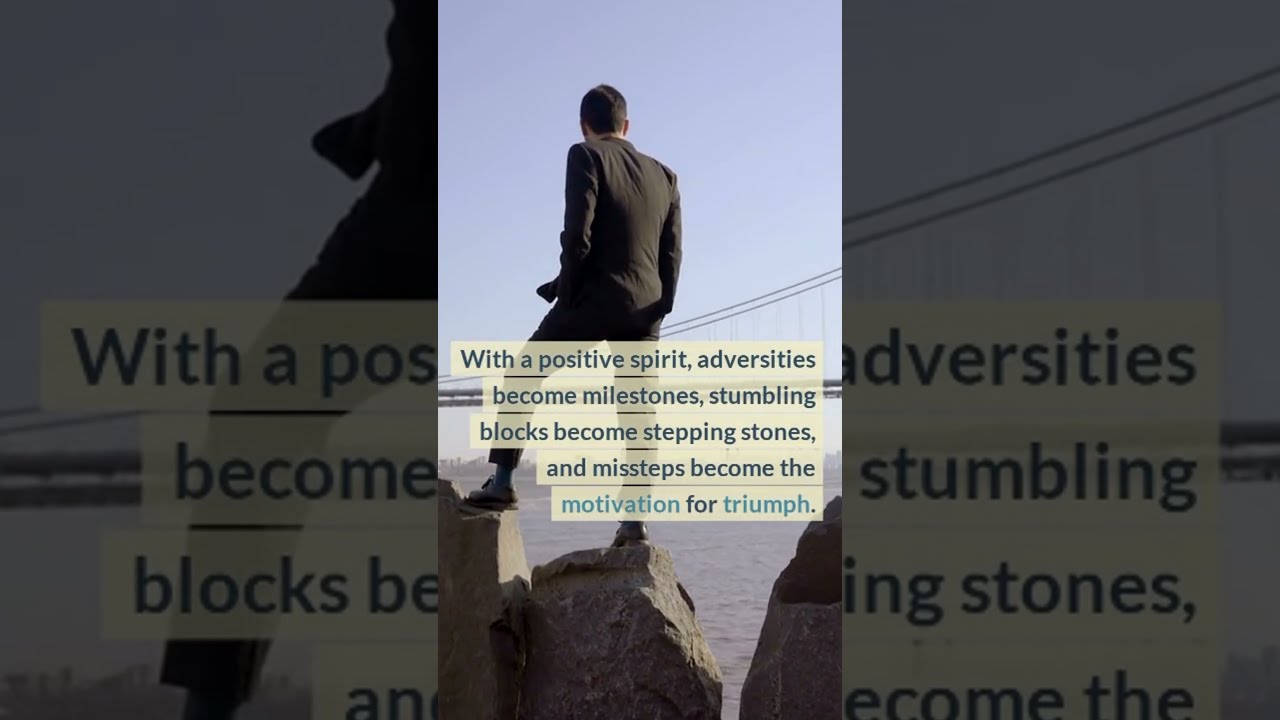The image is a composite of three separate photos featuring the same scene. At the center, a man in a black suit with short dark hair is standing on uneven boulders, with one foot higher than the other, facing away from the camera. His hands appear to be in his pockets. He is gazing towards the Golden Gate Bridge, which is prominently visible against a pale blue sky. Below the bridge, there is a body of gray, slightly rippling water. 

The central photo shows the man fully, surrounded by text in yellow banners with dark letters that reads: "With a positive spirit, adversities become milestones, stumbling blocks become stepping stones, and missteps become the motivation for triumph." 

The left and right sections of the composite image are filtered and grayed-out enlargements of parts of the central photo. The left section shows just his leg and coat tails, while the right section highlights fragments of the text, with words like "adversities," "stumbling," and partial phrases such as "ing stones" and "ecum the" visible. The natural daylight illuminates the scene, emphasizing the contemplative and motivational theme of the image.